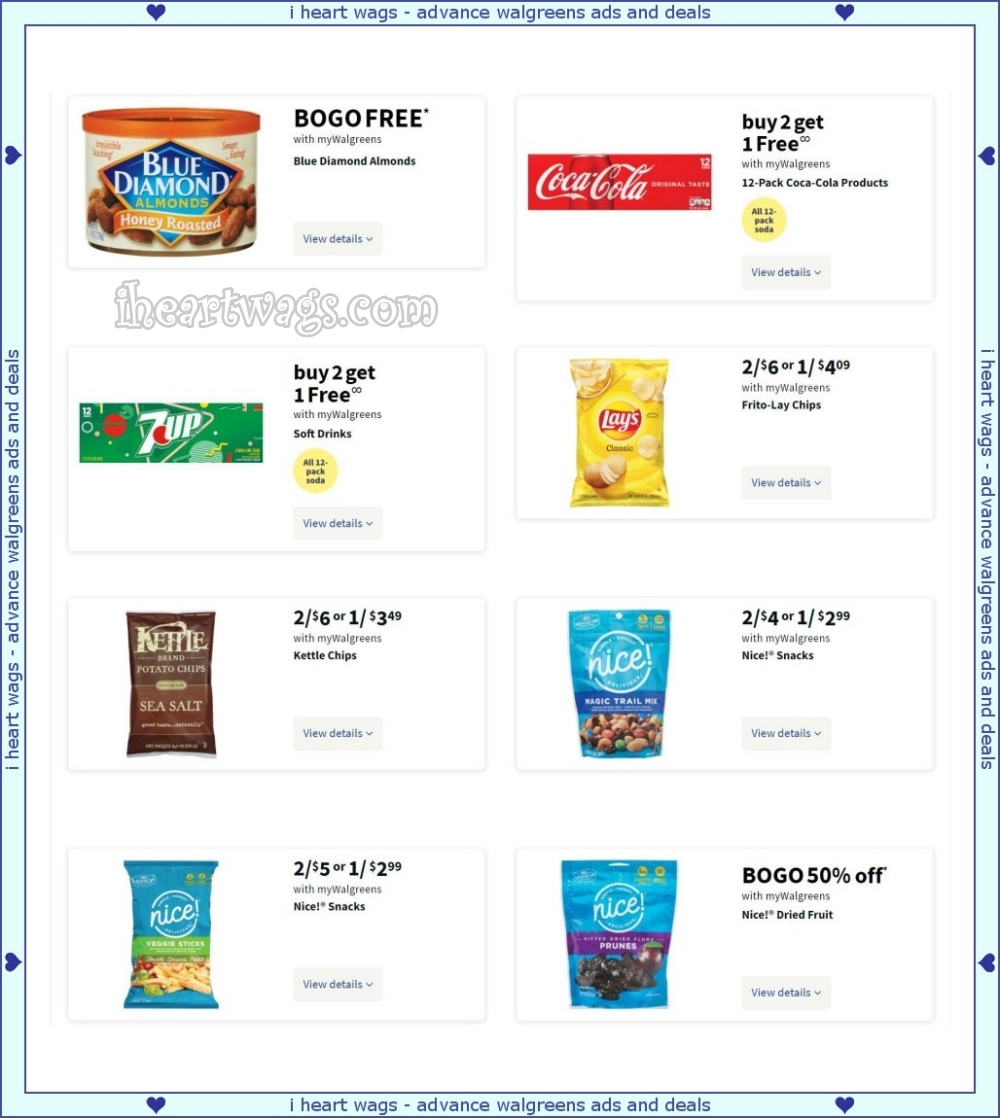The image features a visually appealing web page with a border consisting of light blue with a darker blue trim, adorned with little blue heart icons. Prominently displayed at the top is the text, "I ♥ Wags – Advance Walgreens Ads and Deals," indicating a collection of special offers at Walgreens. The web page showcases various deals, each accompanied by a "view details" link. 

Highlighted deals include:
- Blue Diamond Almonds in cans: Buy one, get one free with myWalgreens membership.
- Coca-Cola products: Buy two 12-pack, 12-ounce cans and get one free.
- 7 Up products: Buy two, get one free.
- Frito-Lay chips: Two for $6 or one for $4.09.
- Kettle Chips: Two for $3 or one for $3.49.
- Nice brand snacks, including trail mix: Two for $4 or one for $2.99.
- Nice brand veggie sticks and dried fruit, including prunes: Buy one, get one free.

At the bottom-left corner, a small link to "iheartwags.com" is visible. The arrangement and design focus on promoting value deals to engage shoppers at Walgreens.